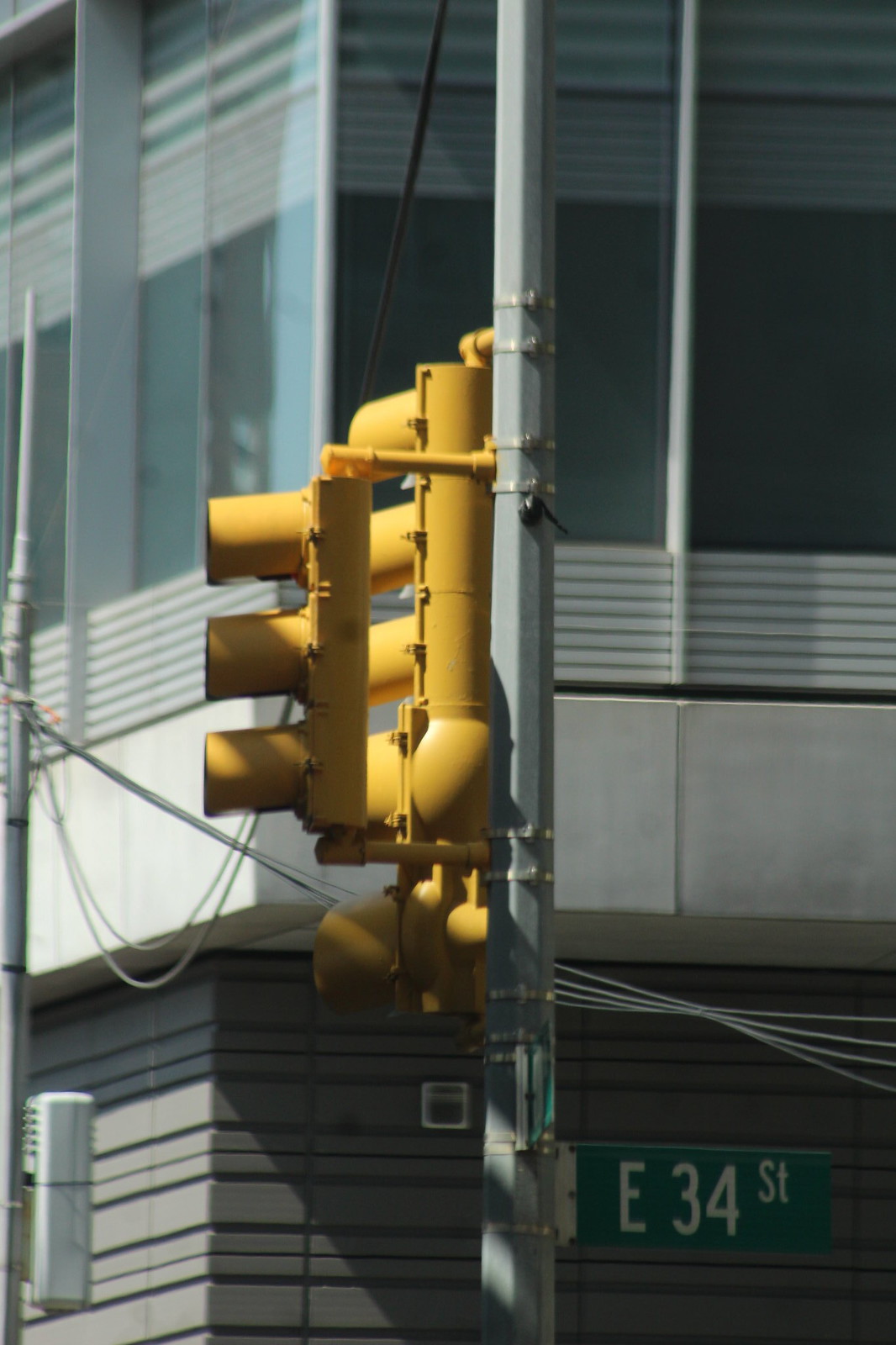The image depicts a street scene featuring a prominent yellow traffic light. The light has three bulbs encased in a yellow housing and is attached to a tall, rectangular metal pole that has an octagonal shape. A green rectangular sign reading "E 34th St" in white lettering protrudes from the bottom right of the pole. The background showcases a large building, which could be either a corporate or apartment complex. The building features transparent yet very dark windows bordered by long, light gray panels. Below these windows, there is a cement structure. A collection of traffic lights is visible in front of the building, with one light featuring four bulb casings and another displaying a larger single bulb casing, all in a mustard yellow color. The pole with the three-bulb light extends upward, with a black nub near the top middle from which a string appears to dangle. The scene lacks visible sky, dominated entirely by the building facade, and exudes an urban atmosphere.